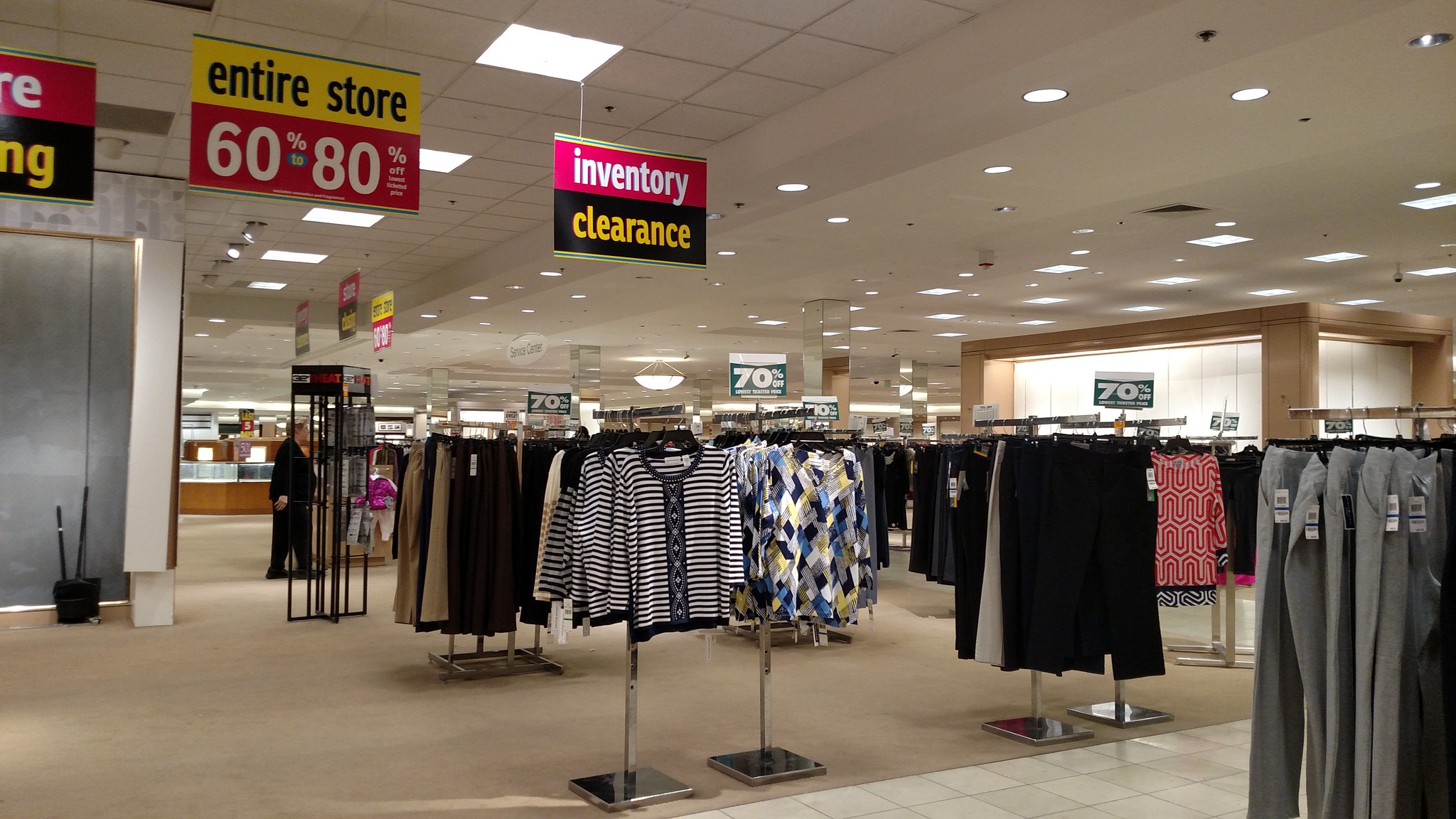This photo captures the interior of a department store amidst an inventory clearance sale. The beige carpeted floor lends a soft contrast to the array of clothing racks filled with pants and shirts. To the left, a sleek silver elevator is visible. The ceiling comprises white rectangular tiles, illuminated by a combination of square fluorescent lights and recessed canister lights.

Signs are prominently displayed, announcing significant discounts ranging from 60-80% off as part of a storewide closing sale. Above one clothing rack, a sign specifically advertises a 70% off discount, indicating that this section likely pertains to women's apparel. In the background, a woman dressed in a black pantsuit is seen walking, adding a human element amidst the retail setup. The image encapsulates the final days of a department store, bustling yet imbued with a sense of conclusion.